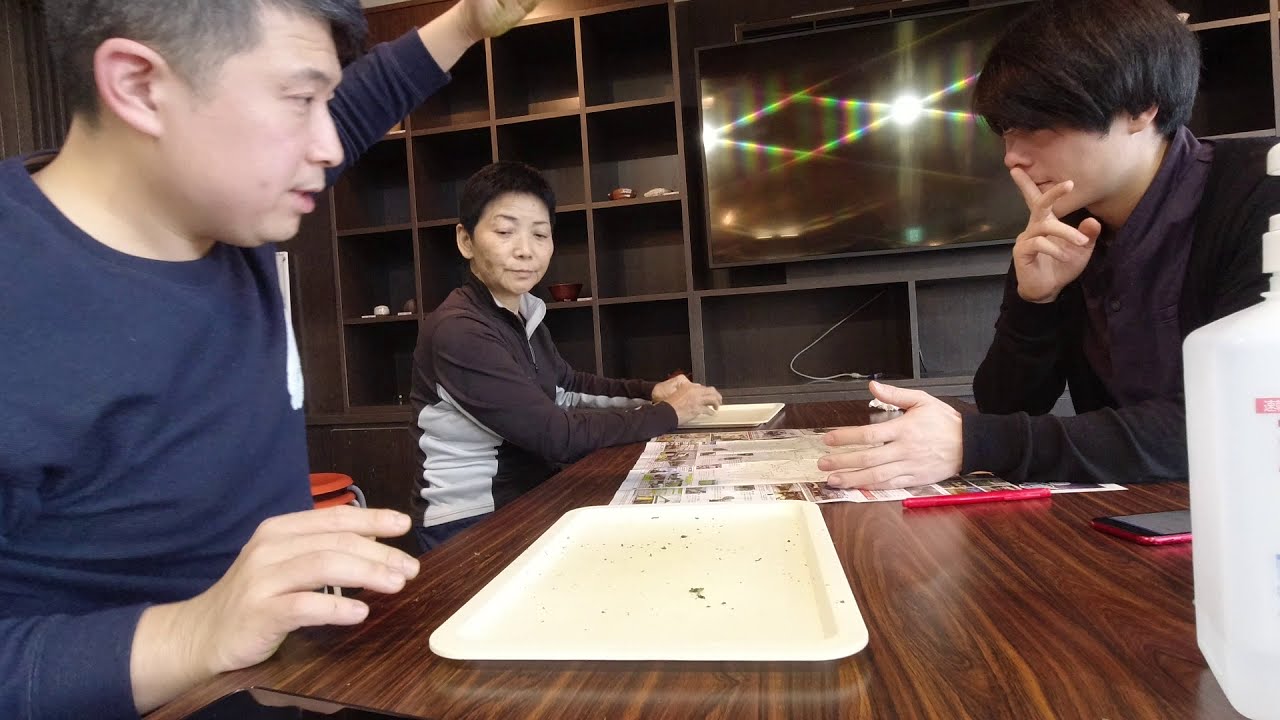In a cozy room that appears to be a library, three Asian individuals sit around a brown wooden table, engaged in what seems to be a board game. At the table's forefront, capturing the left-hand side of the picture, a man with a pointed ear and short, straight black hair is prominently featured. Dressed in a dark blue long-sleeved crew-knit shirt, he raises his left hand while resting his right hand on the table, seemingly looking towards his opponent across the table.

Beside him sits a woman with short straight black hair, clothed in a long-sleeved brown shirt adorned with vertical white stripes. She is attentively glancing towards the first man's direction.

Across from them sits a younger man with long black hair partially covering his eyes. He rests his right elbow on the table, his right index finger raised to his mouth in a "shh" gesture, as if contemplating his next move or advising quietness. His left hand is splayed out on the table.

In front of this contemplative man lies a white rectangular tray or mat, and some kind of board game that includes pieces and potentially a paper with writing or images. The background of the scene features bookshelves and a television, adding to the library-like ambiance.